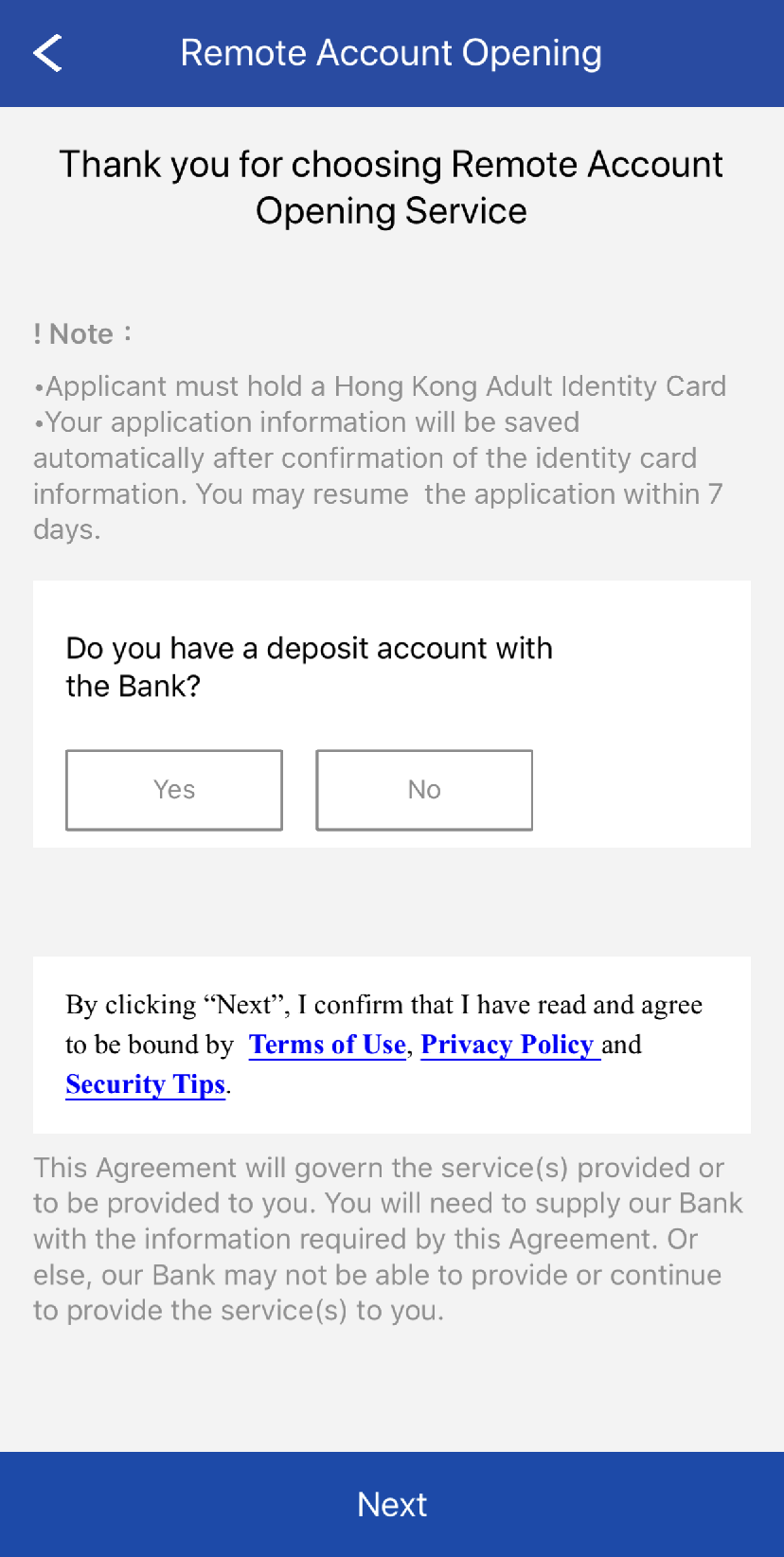The image depicts the user interface for a remote account opening service. At the top center, a prominent blue banner displays the title: "Remote Account Opening." Directly beneath the banner, bold text reads, "Thank you for choosing our remote account opening service."

Following this, a section labeled "Note" appears in a lighter gray font. The note specifies important requirements and instructions: "Applicant must hold a Hong Kong adult identity card. Your application information will be saved automatically after confirmation of the identity card information. You may resume the application within seven days."

Below the note, a white box with black text asks, "Do you have a deposit account with the bank?" Accompanying this question are two selectable options, "Yes" and "No," each encapsulated in distinct blocks.

Further down the page, another white box contains the following disclaimer in black font: "By clicking 'Next,' I confirm that I have read and agree to be bound by the Terms of Use, Privacy Policy, and Security Tips."